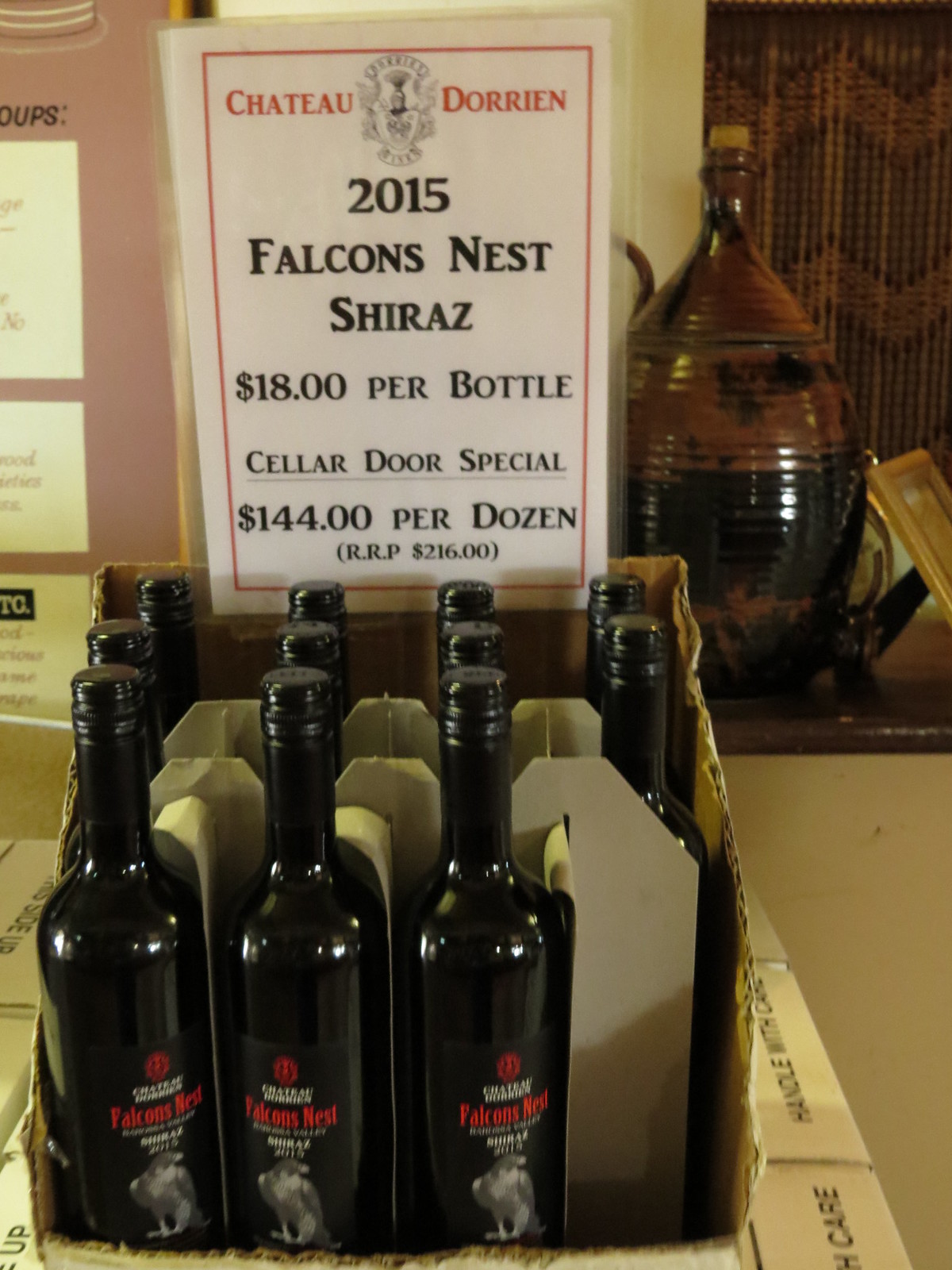This photograph captures an indoor, low-light scene featuring a partially torn cardboard box arranged in a three-by-four grid, revealing 11 black glass bottles of wine with red and white labeling. The labels prominently feature the text "Falcon's Nest" while additional details are blurred. A single bottle is missing from the lower right section of the box. Behind the box, a laminated sign on white paper with a red border advertises the wine, reading: "Chateau Dorian, 2015 Falcon's Nest Shiraz, $18 per bottle, Cellar Door Special $144 per dozen, RRP $216." The background includes an off-white or yellow wall adorned with additional signage, a brown jug, a picture frame on a countertop, and a beaded brown curtain in the far right corner, suggesting a contextual setting that could be a wine store or a section within a restaurant.